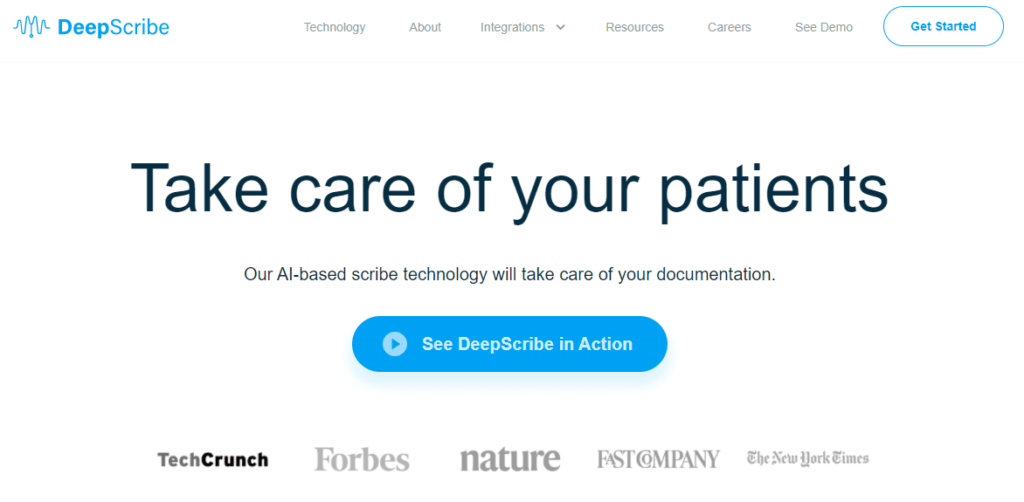The image is a horizontal screenshot of a webpage with a clean white background and no border. In the upper left-hand corner, the company's logo and name, "DeepScribe," are displayed. The logo consists of a blue squiggle adjacent to the company's name written in a blue font. To the right of the logo, there are several header drop-down menus labeled Technology, About, Integrations, Resources, Careers, and C-Demo. 

In the upper right-hand corner, there is a blue outlined button with the text "Get Started." Dominating the center of the image is a prominent heading in large black font that reads "Take Care of Your Patients." Beneath this, in smaller font, a subheading states, "Our AI-Based Scribe Technology Will Take Care of Your Documentation."

Just below this text, there is a horizontal light blue bubble featuring an arrow icon that indicates it can be clicked to play a video. The bubble contains the text, "See DeepScribe in Action." 

At the bottom of the image, the logos of five different companies are displayed in their characteristic fonts, from left to right: TechCrunch, Forbes, Nature, Fast Company, and The New York Times. The webpage is aimed at promoting Scribe Technology, and viewers can click the central button to learn more about the technology.